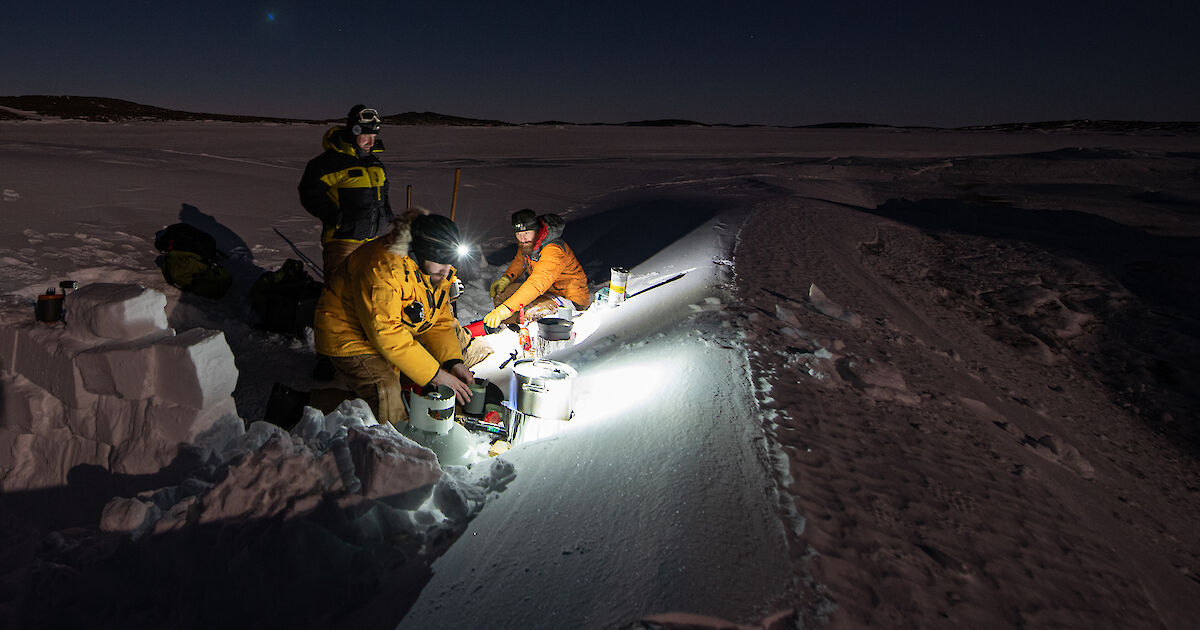In this captivating photo of a wild, natural setting, we see a vast, icy landscape bathed in a reddish hue, likely due to the unique lighting conditions. The wide, dusty expanse stretches out under a darkening sky, creating an eerie yet fascinating ambiance. In the foreground, three men, possibly more, are engaged in cooking and setting up camp. They are possibly researchers or explorers, dressed in heavy coats, hats, hoods, and helmets equipped with lights. One man stands out, working without gloves amid the harsh environment. Behind a small hill for some shelter, they've constructed an igloo-like structure from ice blocks, providing a temporary refuge in this immense, snowy wilderness. The scene captures the rugged beauty and the challenges of surviving in such a remote, icy expanse.